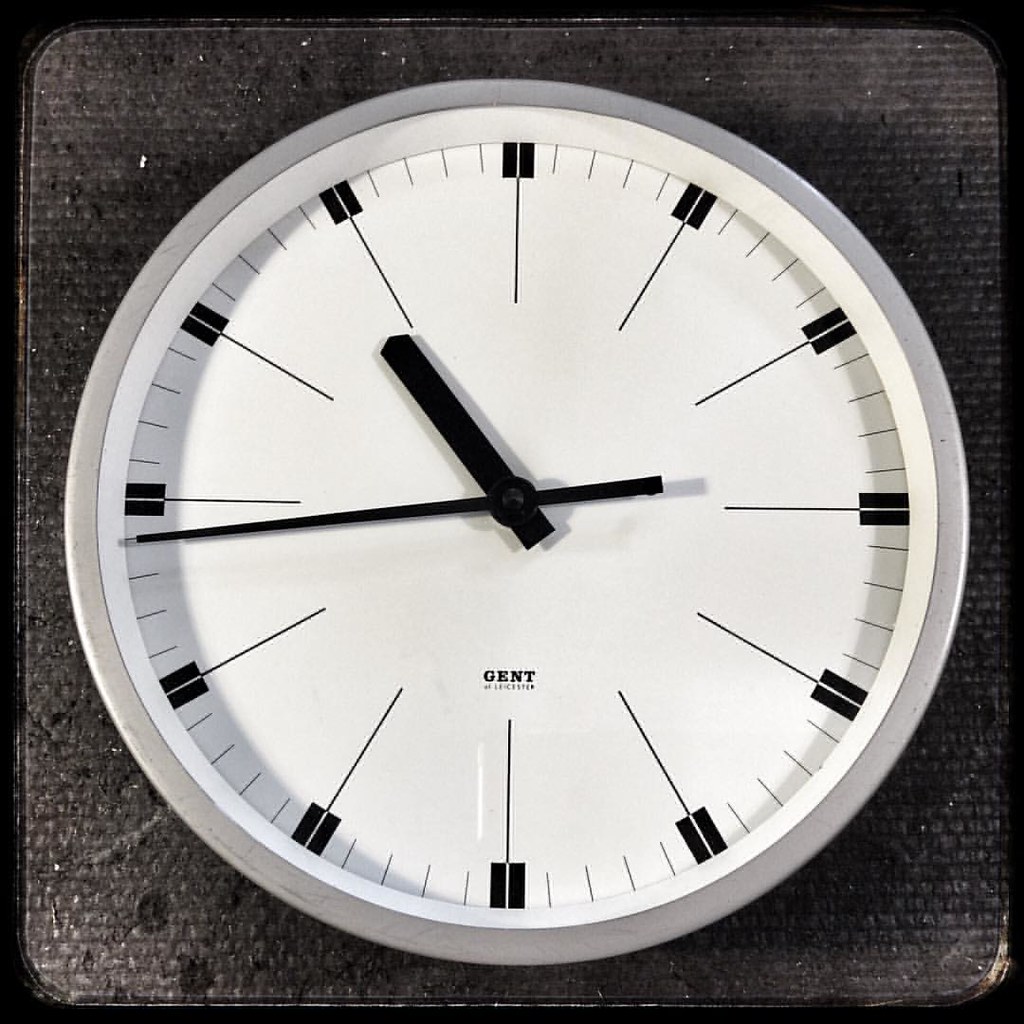This artwork depicts a meticulously detailed clock. The outermost edge features a jet black border, adding a striking contrast to the overall composition. Inside this border is another black box, colored with a dull, shaded black and further accentuated by a darker black outline, creating a sense of depth and dimension.

The clock itself boasts an elegant design with an outer silver border, followed by an inner gray border. The clock's face is pristinely white, enhancing the visibility of its unique markers. Instead of traditional numbers, it has straight black lines representing each hour, with small solid black boxes positioned near the gray border for additional emphasis. Between these hour markers, there are subtle gray lines denoting the minutes.

The minute and hour hands of the clock are also stark black, standing out prominently against the white background. The detailed contrasts and precise markings reflect a sophisticated and modern interpretation of timekeeping.